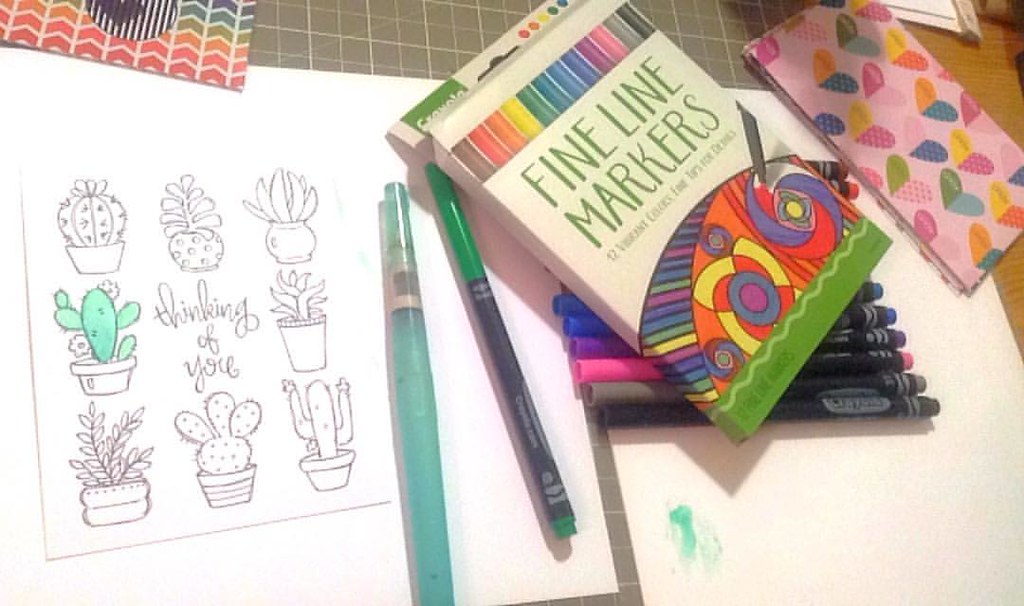The image depicts a detailed scene of an art station set up on a brown veneer desk. Central to the image is a white piece of paper sectioned into grids, featuring pencil outline drawings of various cute cactuses, some of which look like they are in little pots and one resembling a cowboy. The cactuses circle around the scripted words "Thinking of You." One cactus has been colored in a light green, with only the flowers remaining uncolored. To the right of the paper lies a box of 12 fine line markers, showcasing a spectrum of colors from black to cream. Some markers are scattered on the desk, while the box tops them. Additionally, there are crayons and an object with hearts that resembles a checkbook, adding to the colorful and artistic nature of the scene.